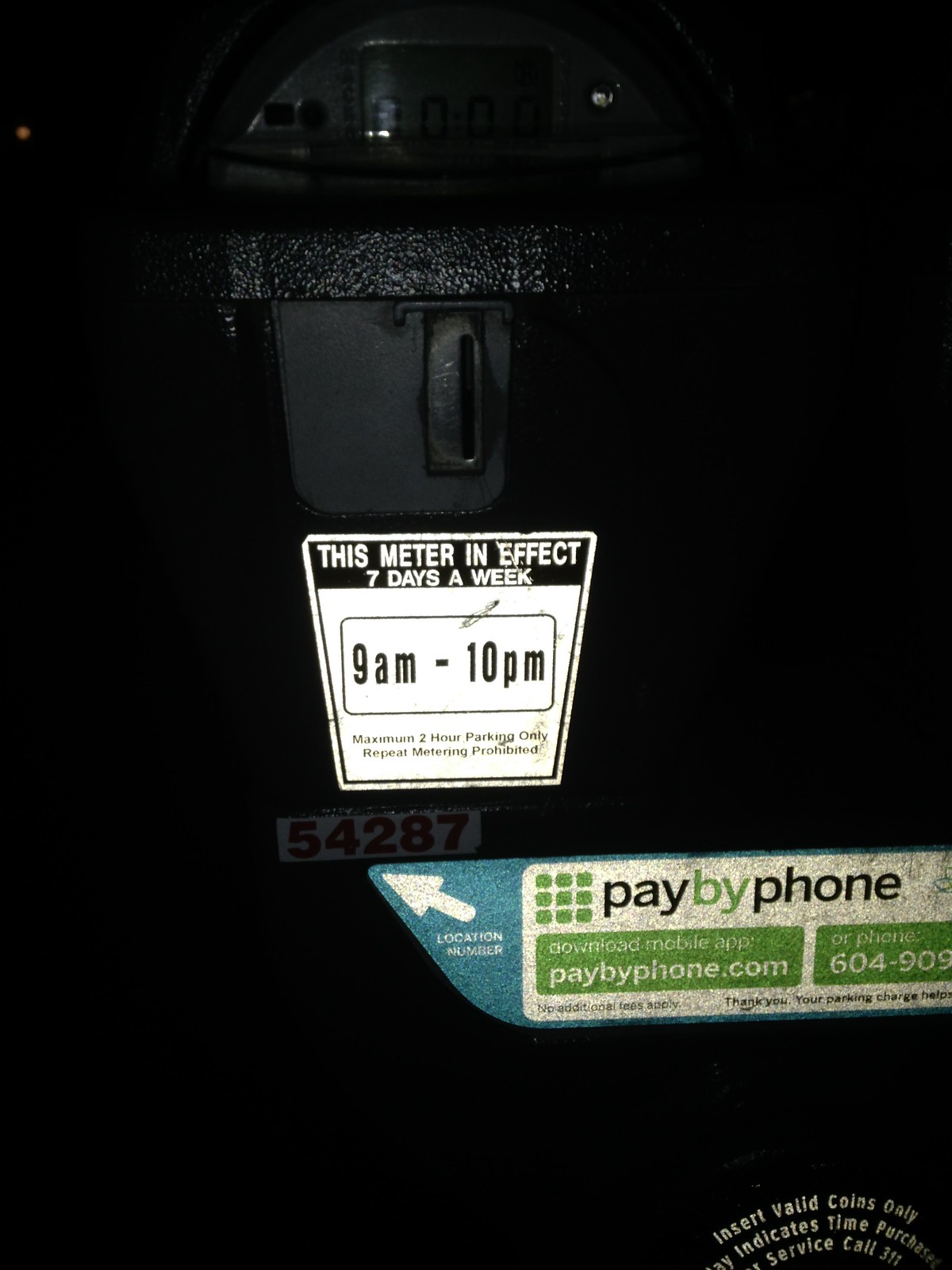The image shows a close-up of an old-fashioned, metal parking meter, partially illuminated against a very dark, nighttime background. The top of the parking meter features a slot for inserting coins and is adorned with a couple of stickers that stand out. The primary sticker, white with black text, reads "This meter is in effect 7 days a week, 9am to 10pm" and "Maximum 2-hour parking only, repeat metering prohibited." Below this is a rectangular sticker shaped like half a canoe, promoting a "pay by phone" option. This sticker includes a web address, paybyphone.com, and a partially visible phone number preceded by "604." Additionally, there's a noticeable detail of a red location number "54287" highlighted by a shiny turquoise arrow. The text and arrows are in various colors, with "pay" in black, "by" in green, and "phone" in black, complemented by green dots and areas. Further text indicates information about downloading a mobile app, inserting valid coins, and contacting service via 311, although some of these details are obscured.